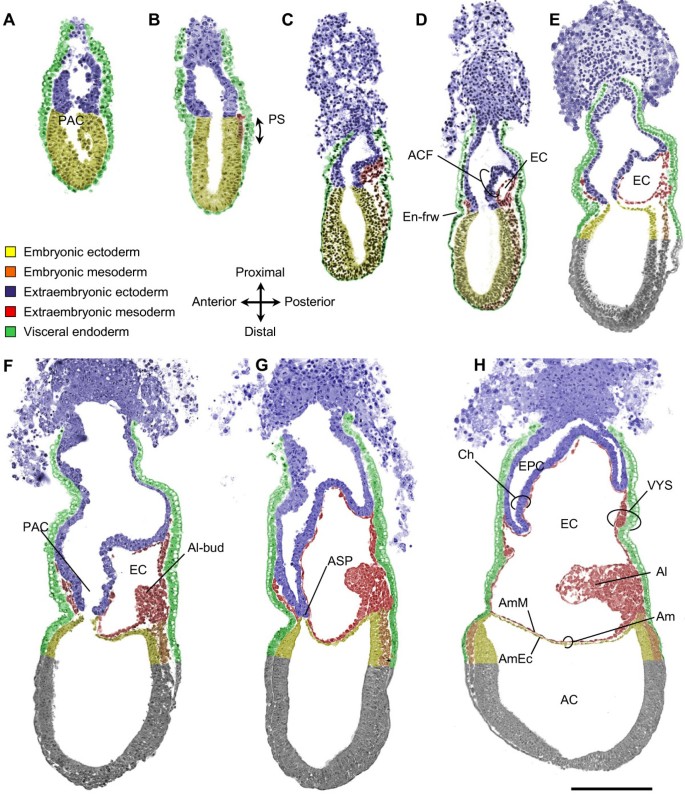This detailed image from a scientific textbook or educational material depicts eight cellular organisms arranged in a two-part diagram. The upper part, labeled from A to E from left to right, shows progressively larger and diversified cells. The lower part, lettered F to H, continues this trend with even larger and more detailed cells. Each organism is depicted in distinct colors, including green, purple, yellow, and red, indicating different cellular components. The diagram includes a compass-like indicator, with labels for proximal (top), posterior (right), distal (bottom), and anterior (left). Additionally, a color-coded guide provides further explanations: yellow for embryonic ectoderm, orange for embryonic mesoderm, blue/purple for extraembryonic ectoderm, red for extraembryonic mesoderm, and green for visceral endoderm. The organisms exhibit a pattern with smaller cells on the top row, increasing in size towards the bottom row, enhancing the educational value of the image.